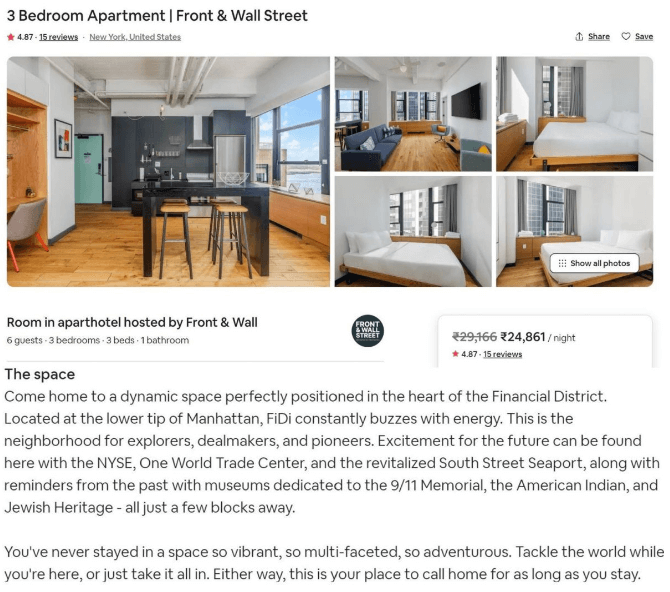**Luxurious Three-Bedroom Apartment in New York's Financial District**

This captivating listing showcases a luxurious three-bedroom apartment located at the intersection of Front and Wall Street in the heart of New York City's vibrant Financial District. Rated 4.87 out of 5 stars based on 15 reviews, this exquisite accommodation offers unparalleled comfort and style, ideal for explorers, deal-makers, and pioneers alike.

The apartment, hosted by Front and Wall, is designed to accommodate up to six guests. It features three beautifully furnished bedrooms, each with its own bed and window, ensuring ample natural light and serene views. The living room is tastefully appointed with a plush couch, sofa, TV, and chairs, creating an inviting space for relaxation. The spacious kitchen and dining area are perfect for culinary adventures and enjoying meals with loved ones.

As of the current promotion, the pricing for this exclusive accommodation has been reduced from $29,166 to $24,861 per night. In addition to the stunning visuals of the apartment, the listing includes a share button and a save button for convenient browsing and future reference.

Nestled at the southern tip of Manhattan, this dynamic space is perfectly positioned to experience the constant buzz and energy of the Financial District. The neighborhood is an exciting mix of the old and new, with landmarks like the New York Stock Exchange (NYSE), One World Trade Center, and the revitalized South Street Seaport showcasing the area's significance in the past and present.

For those interested in cultural and historical exploration, the apartment is just a few blocks away from the 9-11 Memorial museums, the National Museum of the American Indian, and the Museum of Jewish Heritage. This vibrant and multifaceted location offers endless opportunities for adventure and discovery.

Whether you plan to tackle the world or simply take in the atmosphere of one of New York's most iconic neighborhoods, this exceptional apartment is the perfect place to call home during your stay.